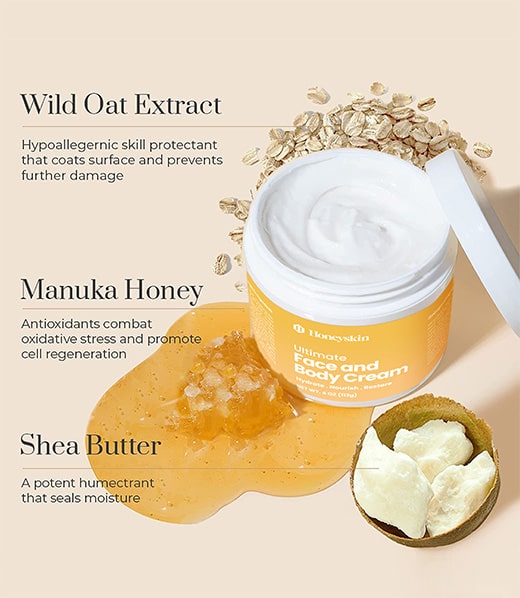On a pale beige background, a meticulously arranged scene showcases a jar of face and body cream prominently displayed with its white lid unscrewed and revealing smooth, white cream inside. The jar features an orange label with white text. Surrounding the jar, you can see raw ingredients: oats scattered around the top, a pool of honey at the bottom, and shea butter pieces in a small container to the side. Annotations in black text on the left describe the product's key ingredients and benefits: "Wild Oat Extract - hypoallergenic skin protectant that coats the surface and prevents further damage," "Manuka Honey - antioxidants combat oxidative stress and promote cell regeneration," and "Shea Butter - a potent humectant that seals moisture." This detailed setup not only highlights the product but also emphasizes the natural, beneficial ingredients used in its formulation.